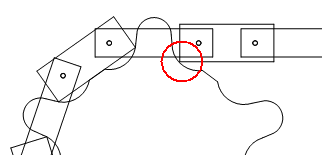This image, reminiscent of digital art created in a simple application like Paint, features a minimalist pattern composed of variously sized rectangles. Starting from the bottom left corner, where a connection is implied but not visible, the rectangles progressively overlap upward diagonally towards the right. Each overlapping segment is connected by a small circle, resembling a bolt, providing a sense of continuity and connection throughout the pattern. The rectangles vary, transitioning from skinnier, longer shapes to thicker, shorter ones.

A squiggly line weaves through the entire pattern, adding a dynamic element to the otherwise linear composition. At the central intersection, where two rectangles meet and the squiggly line crosses, a prominent red circle highlights this focal point, drawing attention to both the intersection of the rectangles and the squiggly line. The pattern then shifts direction, extending horizontally to the right with more overlapping rectangles, each segment also marked by the small circular 'bolts'. This clean yet intricate composition blends geometric precision with a touch of spontaneity from the squiggly line, creating a visually engaging piece.